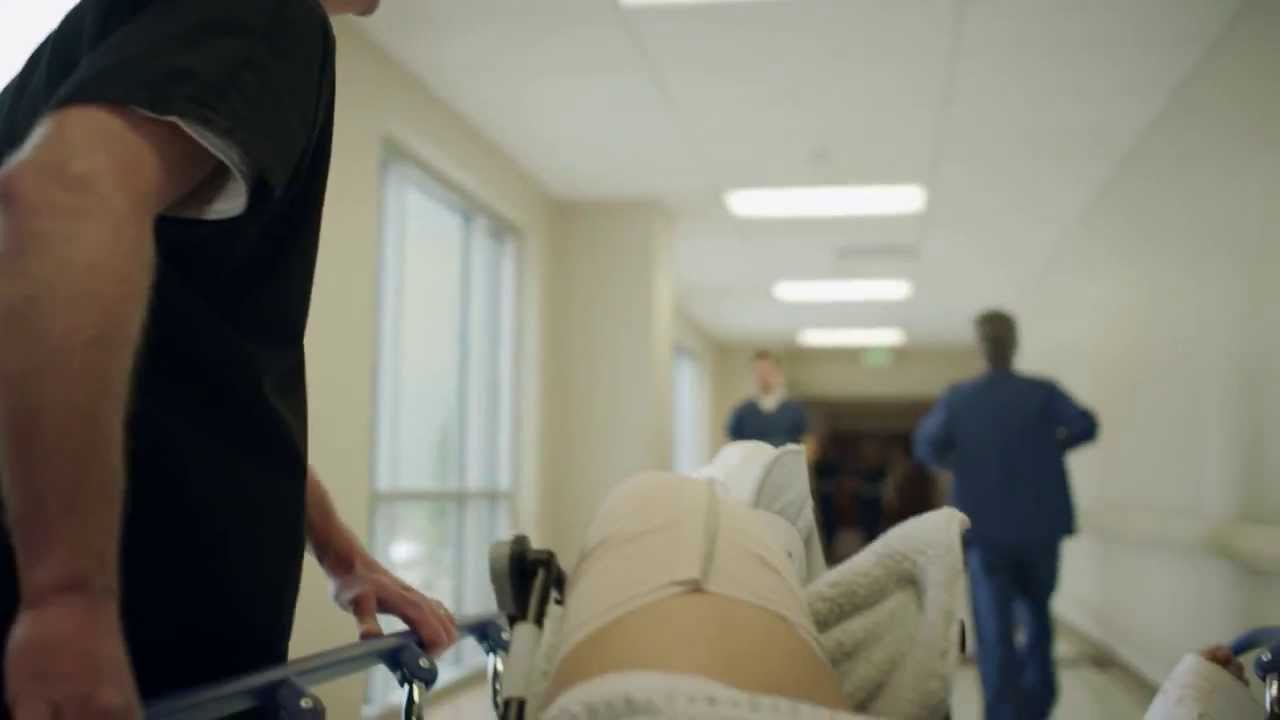This detailed photograph captures a hospital scene from the point of view of a patient being transported on a gurney. The image focuses on the patient's legs, with the right leg propped up and wrapped in an ace bandage and possibly a plaster cast visible in the bottom right corner. An orderly, dressed in dark blue scrubs with a short-sleeve white shirt underneath, is pushing the gurney from the left side, his hands gripping the rail. The background reveals a long, white hallway with large windows to the side, filled with other medical staff, slightly out of focus. Two individuals are walking in the corridor; one, in similar blue scrubs, is heading towards the gurney, and the other, wearing a blue suit, is walking away. The ceiling is equipped with horizontally placed fluorescent lights at regular intervals, and the walls are cream-colored, adding to the clinical ambiance of the scene.